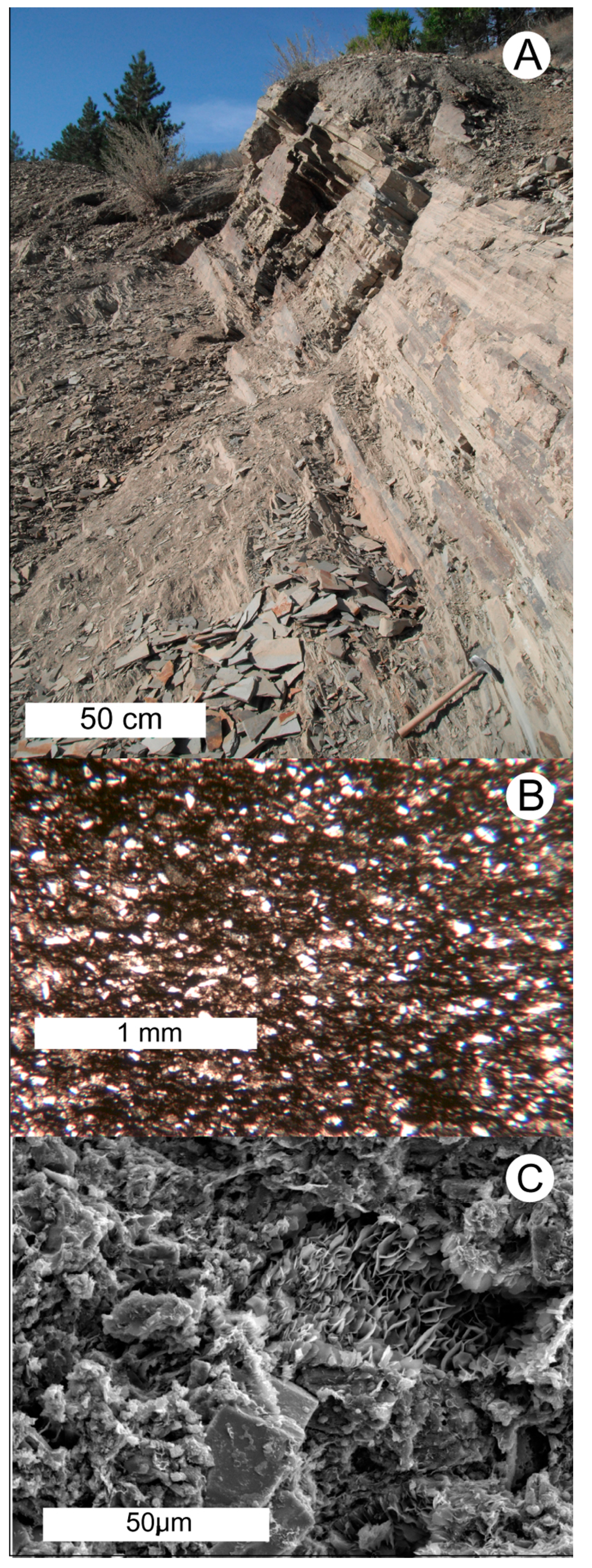This composite image consists of three vertically-stacked photographs showcasing different magnifications of a cliffside composed of shale and thin rock layers. 

The top photograph features a broad view of the cliffside, marked by a hammer for scale, with layers of brown rock. In the top right corner, a large white circle with a black letter 'A' is visible, while the bottom left corner has a white rectangle with black text reading "50 cm" indicating the scale.

The middle photograph zooms in on the cliffside, revealing a detailed view of brown rock interspersed with numerous white dots. A black letter 'B' within a white circle can be found in the top right corner, and a white rectangle with "1 mm" in black text is located in the bottom left, denoting the scale.

The bottom photograph offers an even closer, presumably microscopic view of the rock, shown in green hues with various shapes visible. The top right corner features a black letter 'C' within a white circle, and the bottom left corner displays a white rectangle with the text "50 μm" in black, representing the microscopic scale.